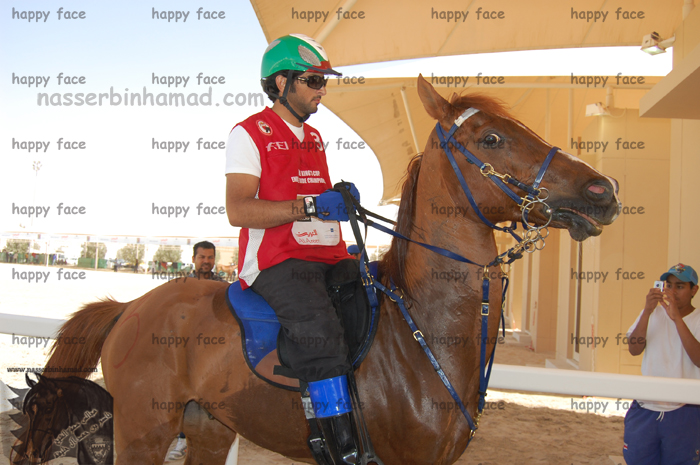In the image, a brown horse appears slightly scared as it stands still, viewed from its right side, looking towards the camera. A rider with tanned skin is mounted on the horse, wearing black pants, black boots with blue accents, a red sleeveless shirt over a short-sleeve white undershirt, and a green helmet with a black visor. The horse is equipped with shiny blue reins and a saddle that is black in the front and blue in the rear. In the background, two people are visible, one clearly taking a photo with a phone, wearing a dark blue cap, white short-sleeve shirt, and blue pants, while the other figure is barely discernible. The entire image is overlaid with repeated 'happy face' text in a watercolor-like, copyright watermark fashion, and a URL in the upper left corner reading "nasserbinhamad.com".